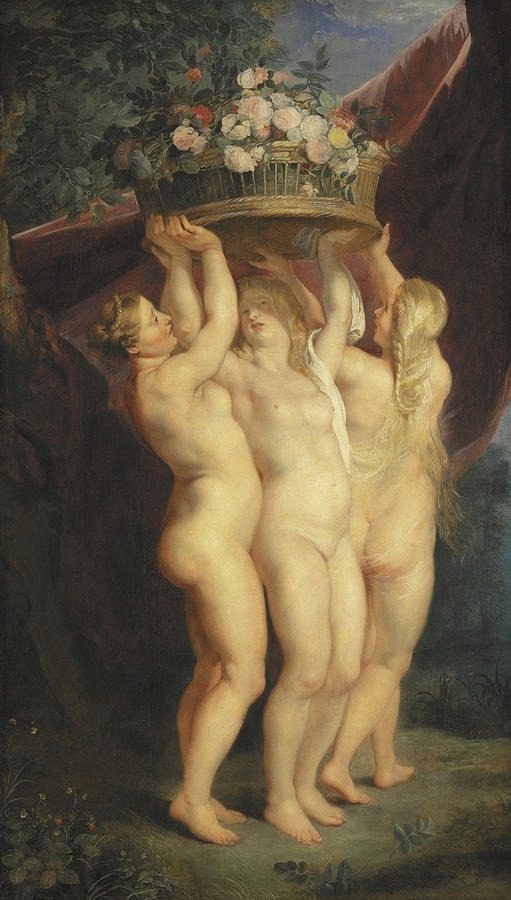The image is a vertically oriented classical painting, possibly from the Renaissance or Romanticism periods, featuring three nude women standing at the center-bottom of the frame. They are depicted in a nature scene, holding up a large, flower-filled vase or basket. The flowers are diverse in color, including pink, blue, red, and yellow roses. Each woman is fairly corpulent and blonde; two have their hair down while the third has her hair done up. All three gaze upwards at the basket they hold aloft. The background includes a small section of blue sky with scattered clouds and a large tree with thick vines and branches on the left side. A possible mountain appears on the right. The painting employs dark and warm colors, contributing to its classical and somewhat somber aesthetic. The women's expressions are neutral, suggesting a potential symbolic burden rather than a depiction of emotional conflict.